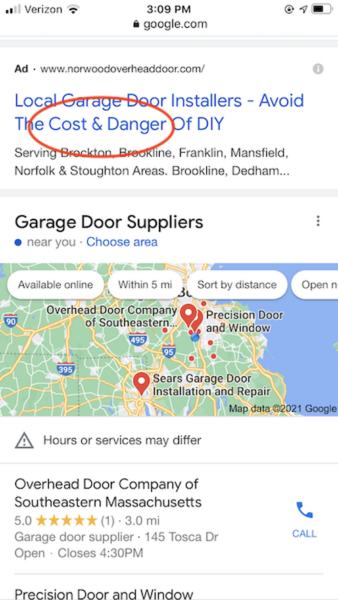A screenshot from an iPhone displays a search for local garage door installers, highlighting the advantages of avoiding DIY efforts. The iPhone status bar at the top shows the time as 3:00 PM, with Verizon as the carrier, and indicates full Wi-Fi signal, active location services, and a fully charged battery. The search appears on the website gober.com. 

A red circle emphasizes the words "cost and danger" to underline the risks associated with do-it-yourself garage door installations. Below the highlighted text, a typical results page presents garage door suppliers. The map accompanying the search results shows various locations for these suppliers.

One of the businesses listed is the "Overhead Door Company of Southeastern Massachusetts," boasting a five-star rating and located three miles away. Additional details include its operational hours and a call icon for direct dialing. Just beneath, the beginning of another business listing, "Precision Door and Window," is visible, but the details are truncated. 

The results layout includes a sponsored section, a local map, and a list of businesses, following the standard format of a Google search page.